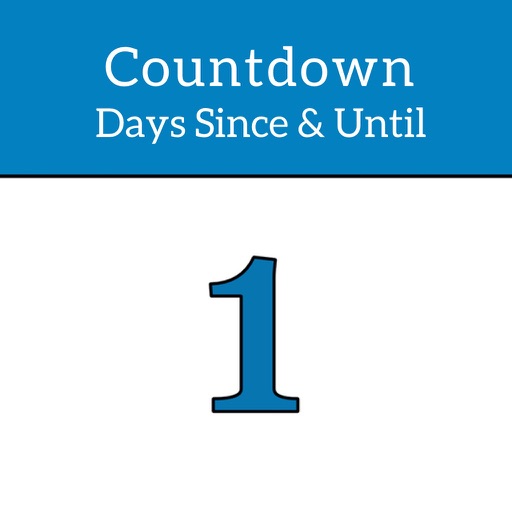The digital image features a countdown calendar design split into two distinct sections. The top 40% of the image has a light blue background with two lines of centered white text: "Countdown" at the top, followed by "Days Since & Until" below it. The text is capitalized and neatly aligned, with the latter phrase slightly deviated to the sides. A thin black dividing line runs horizontally, marking the transition to the bottom 60%, which consists of a plain white background. Centered within this white space is a prominent blue number "1" with a black border outlining it. The number "1" features unique characteristics: its top protrudes and curves downward like a slide, and it has extending feet on both the left and right sides. This clear, computerized layout creates a simple yet effective visual marker commonly used for counting days in various contexts, such as vacation countdowns.